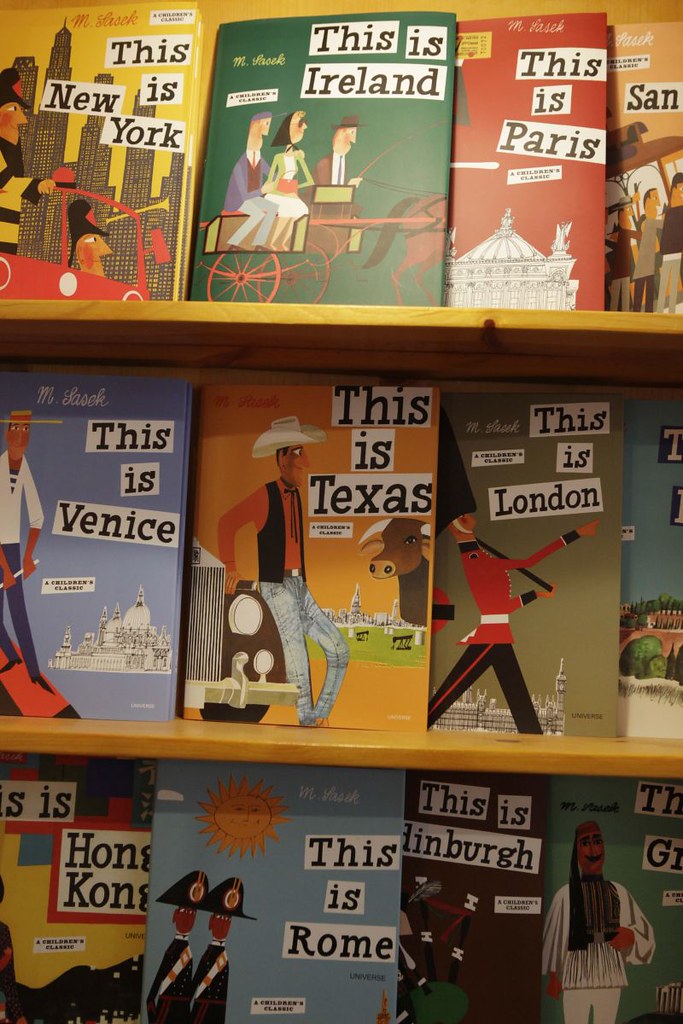The image depicts three yellow wooden bookshelves with a collection of illustrated books prominently displayed, showcasing their covers rather than their spines. Each book is dedicated to a different city or place, featuring vibrant, colorful backgrounds and distinctive illustrations related to each location. On the top shelf, the books are titled "This is New York" with tall buildings, "This is Ireland" with people on a cart, "This is Paris," and a partially visible book with the word "sand." The middle shelf includes titles such as "This is Venice," "This is Texas" with a cowboy and a longhorn bull, "This is London" with a soldier in a bearskin hat, and another book slightly out of frame. The bottom shelf displays "This is Hong Kong," "This is Rome," "This is Edinburgh," and an additional partially visible book starting with a 'G.' Each book appears to be by the same author, given the consistent illustration style featuring characters and scenes pertinent to each place.